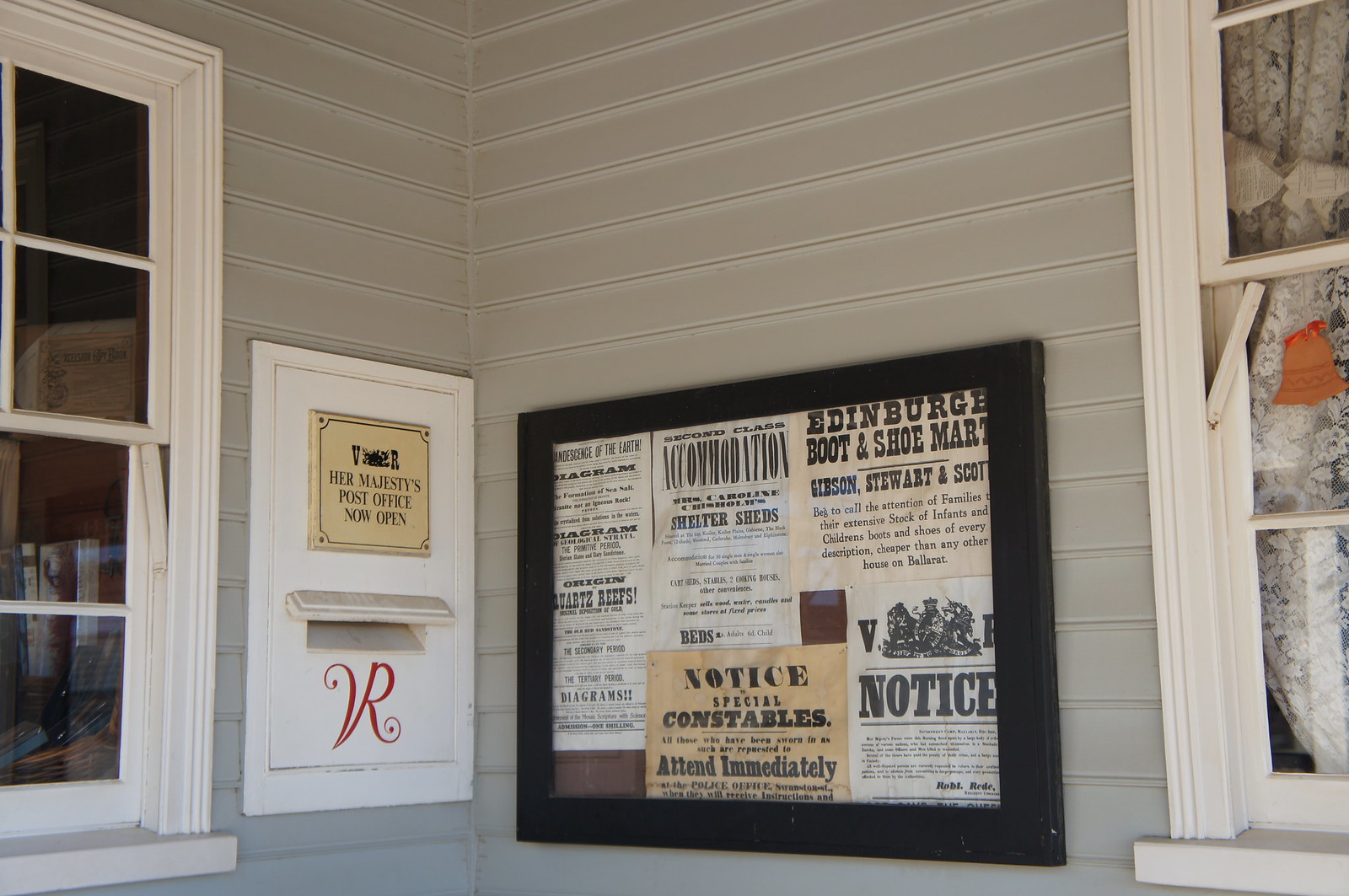This photograph showcases the exterior of a gray, slatted building, possibly functioning as a historical post office. Dominating the center of the image is an intersection of two walls. Prominently placed between two white-framed windows, which are adorned with white lace curtains, is an array of vintage notices encased in a glass-covered board with a black border. The notices include a prominently displayed message reading, "Notice Special Constables Attend Immediately," and another one advertising the "Edinburgh Boot and Shoe Market." Additional notices, some less legible, contribute to the old-world charm. To the left of this noticeboard is an additional prominent feature: a white mail drop slot with the inscription "VR" in red, topped by a gold plaque that declares, "Her Majesty's Post Office, Now Open." The text and overall layout suggest the building's dual purpose as both a residence and a historical business site.